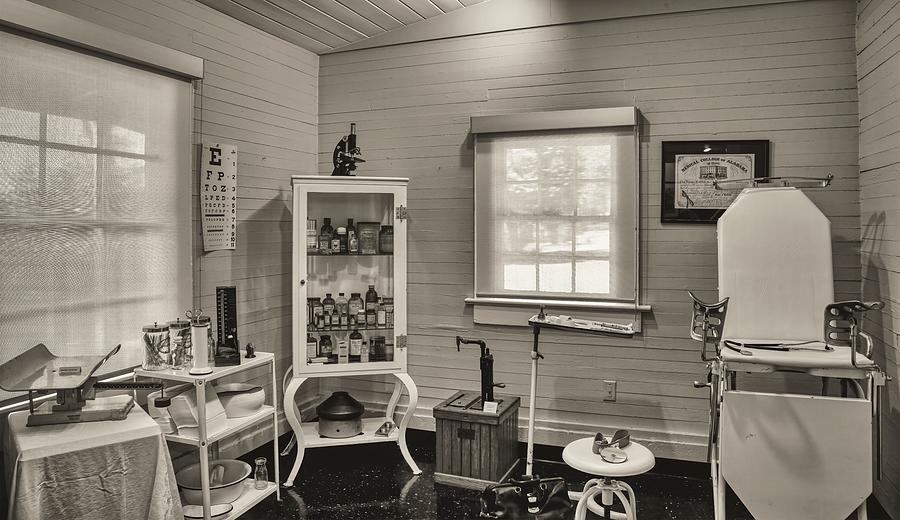The horizontally aligned, sepia-toned photograph captures the inside of a vintage medical room with a detailed layout and various pieces of equipment suggesting its use for medical examinations. Dominating the right side of the room is a distinctive chair with high metal legs, white on one side, featuring metal slots for forearms, and a foldable piece for leg support, likely used for patient exams. Immediate to the chair’s left sits a small white stool on a black and white speckled floor. 

The back wall displays a rich wooden texture with horizontal slats, a window through which a glimpse of trees outside can be seen, and a small rectangular wooden stand beneath the window, possibly containing a faucet. Further left, a wall-mounted eye chart with a prominent capital "E" and smaller letters descending indicates an eye testing area. Above the chart, a magnifying glass is subtly visible.

A white medicine cabinet with a glass door, housing various ointments, bottles, and jars, stands next to the eye chart, with an observable certificate or diploma hanging on one side of the window, adding to the room's clinical authenticity. On the far left, a baby-weighing scale sits on one of the two tables below yet another window. Overall, the room’s wooden walls and antiquated medical furnishing harmonize to create an old-timey, slightly rustic medical parlor ambiance.